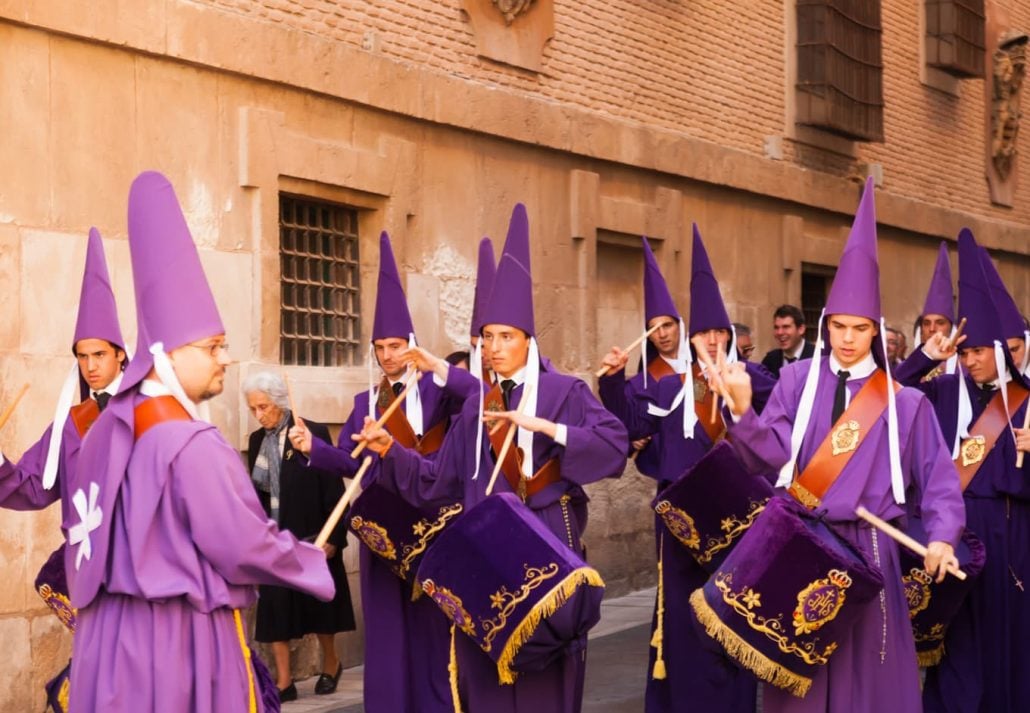In the image, a group of men dressed in elaborate purple robes and tall, cone-shaped purple hats with white tassels are seen marching and playing drums. Each man carries a single drumstick and beats on a large, purple velvet-covered drum adorned with gold tassels and emblems, which is strapped across their chest with a red sash. Their attire includes shirts with white collars and purple ties. Leading the group is a man wearing a similar but slightly lighter purple outfit, who walks backward, ensuring the marchers stay in time, although they appear somewhat disorganized and out of rhythm. To their left, a tan concrete building serves as the backdrop while an older woman in a black suit with a skirt tries to navigate around the group, looking as though she's attempting to avoid them. There is no identifying text, only floral designs in purple on the drums.